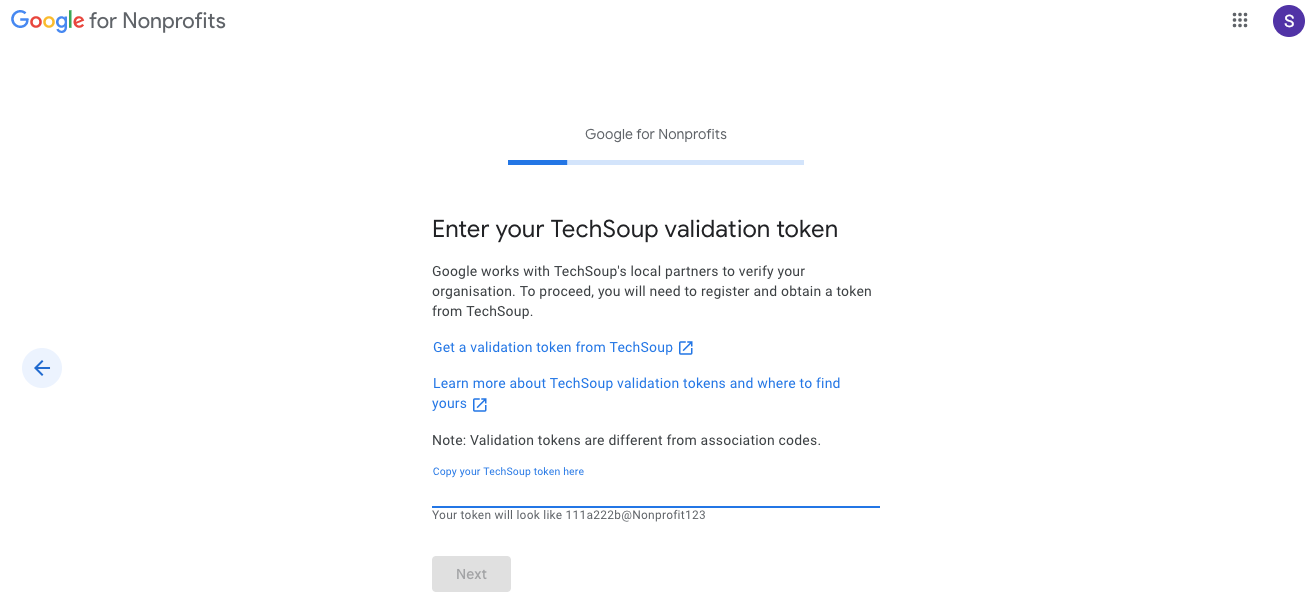This is a screenshot from a website with a white background. In the upper left-hand corner, "Google for Non-Profits" is displayed, with "Google" styled in its iconic logo colors: a blue G, red O, yellow O, light blue O, green L, and red E. The text "for Non-Profits" is in gray. Centrally positioned, the headline "Google for Non-Profits" is repeated, followed by an underlined segment. Most of the underline is a very light blue, while about one-fifth of the left side is in a medium blue. Below this, in gray text, it reads: "Enter your TechSoup validation token. Google works with TechSoup’s local partners to verify your organization. To proceed, you will need to register and obtain a token from TechSoup." A blue-font link underneath says, "Get a validation token from TechSoup," followed by "Learn more about TechSoup validation tokens and where to find yours." At the bottom, a gray note clarifies, "Note: validation tokens are different from association codes."